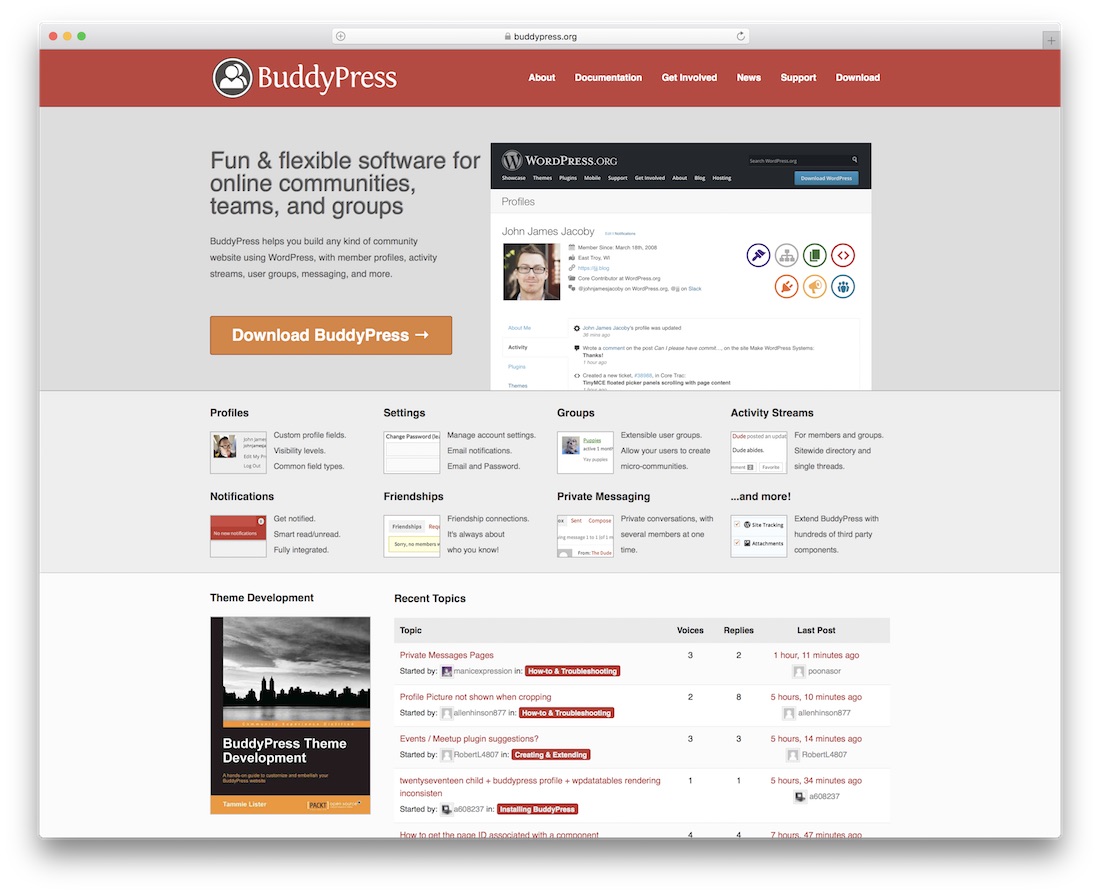The image is a screen capture of the BuddyPress website displayed within a gray-bordered box. At the top of the capture, there are the familiar browser control icons in red, gold, and green. Below this, the white address bar clearly shows the URL: buddypress.org.

Central to the screen is the BuddyPress logo, a black and white circle featuring cartoon characters, accompanied by the text "BuddyPress." Directly beneath are submenus labeled "Documentation," "Get Involved," "Support," and "Download."

Dominating the middle section is a gray box containing a tagline in bold black text: "Fun and flexible software for online communities, teams, and groups." The box elaborates on BuddyPress's functionality, highlighting its integration with WordPress to help build community websites featuring member profiles, activity streams, user groups, messaging, and more. Below this description, there is an orange and white call-to-action button that reads, "Download BuddyPress."

Adjacent to this content, on the right side, is a black and white mock-up of a webpage. This page shows a portrait of a man with brown hair and glasses, identified as John James Jacoby. Surrounding his image are a series of colorful icons in various shades of purple, gray, green, burgundy, orange, and blue.

Further down, another gray box lists clickable links in black text: "Profile Settings," "Groups," "Activity Streams," "Notifications," "Friendships," and "Private Messaging." Each link is accompanied by boxes containing descriptive text and images.

At the bottom of the screen, there is an image of a city skyline in dark hues, overlayed with the text "BuddyPress Theme Development." To the right, there is a section titled "Recent Topics," listing recent discussion topics in red and black fonts. Each topic entry includes details about the voices involved, the number of replies, and the date of the last post.